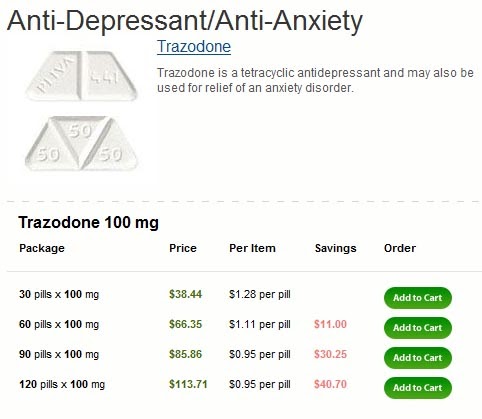**Detailed Caption for Screenshot of Trazodone Listing:**

The screenshot showcases a detailed listing for Trazodone, an antidepressant and anti-anxiety medication, against a white background. The product is a tetracyclic antidepressant often used for anxiety disorder relief, depicted here by an image of two pills labeled as Trazodone 100 mg.

The listing provides several purchasing options for Trazodone 100 mg with the following details:

- **30 Pills:** Total price is $38.44 with a cost of $1.28 per pill. The "Add to Cart" button, displayed in white text on a green oval, is present beneath this option.
  
- **60 Pills:** Total price is $66.35 with a cost of $1.11 per pill, though specific savings are not indicated.
  
- **90 Pills:** Total price is $85.86 with a cost of $0.95 per pill, showing savings of $30.25.

- **120 Pills:** Total price is $113.71 with a cost of $0.95 per pill, showing savings of $40.70.

Each purchase option includes an "Add to Cart" button located in the same green oval format, making it easy for users to select their desired quantity. The listing is informative, clear, and structured to aid potential buyers in making decisions.